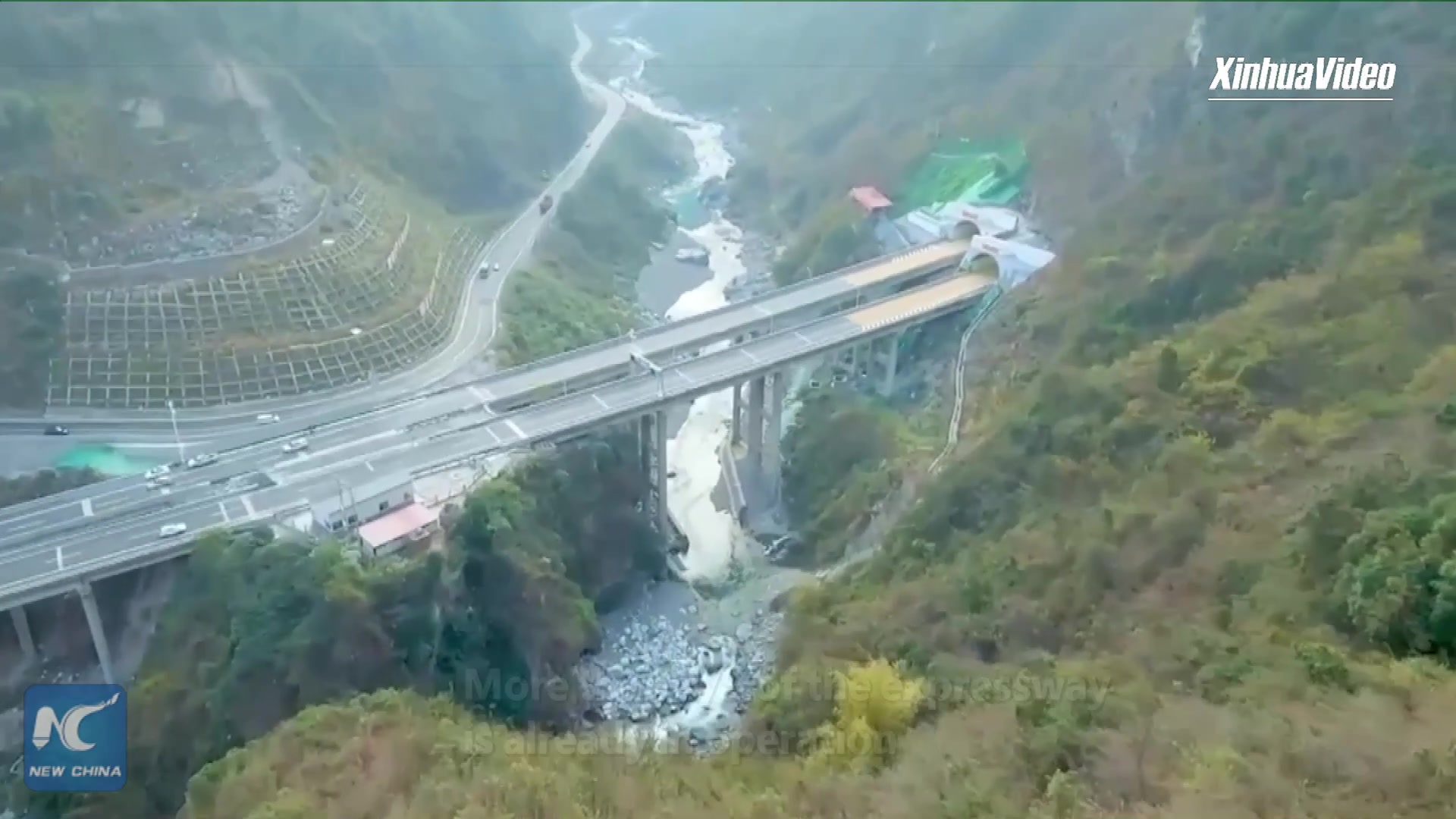This aerial photograph showcases a dramatic and complex mountainous landscape with a bustling highway infrastructure. Dominating the scene are two parallel stretches of a highway intricately designed with a large space in between, creating a precarious bridge-like structure high above a river or stream. The roadway appears to venture into a tunnel carved into a lush, green hillside or grassy mountain. In the foreground, a green tarp is draped over part of the slope, possibly to prevent erosion, and debris, likely dirt, can be seen scattered on the roadway. Vehicles travel both towards and away from the tunnel entrance, adding to the dynamic sense of movement.

To the side of the main highway, another road meanders alongside the waterway, showcasing the extensive and winding nature of the routes carved into this picturesque but seemingly treacherous landscape. Additionally, a constructed wall across the waterway appears to hold back the land, mitigating the effects of erosion during heavy rain. Despite the blur and distance of the image, the lush greenery of the mountain is evident, enhancing the natural beauty of the scene.

In terms of textual elements, the upper right corner of the image displays the text "Xinhua Video," indicating the source, while the lower-left corner features a blue square logo with the words "NC New China." The image captures the intricate balance of human engineering and natural landscape, presenting both the beauty and potential dangers inherent in such an environment.